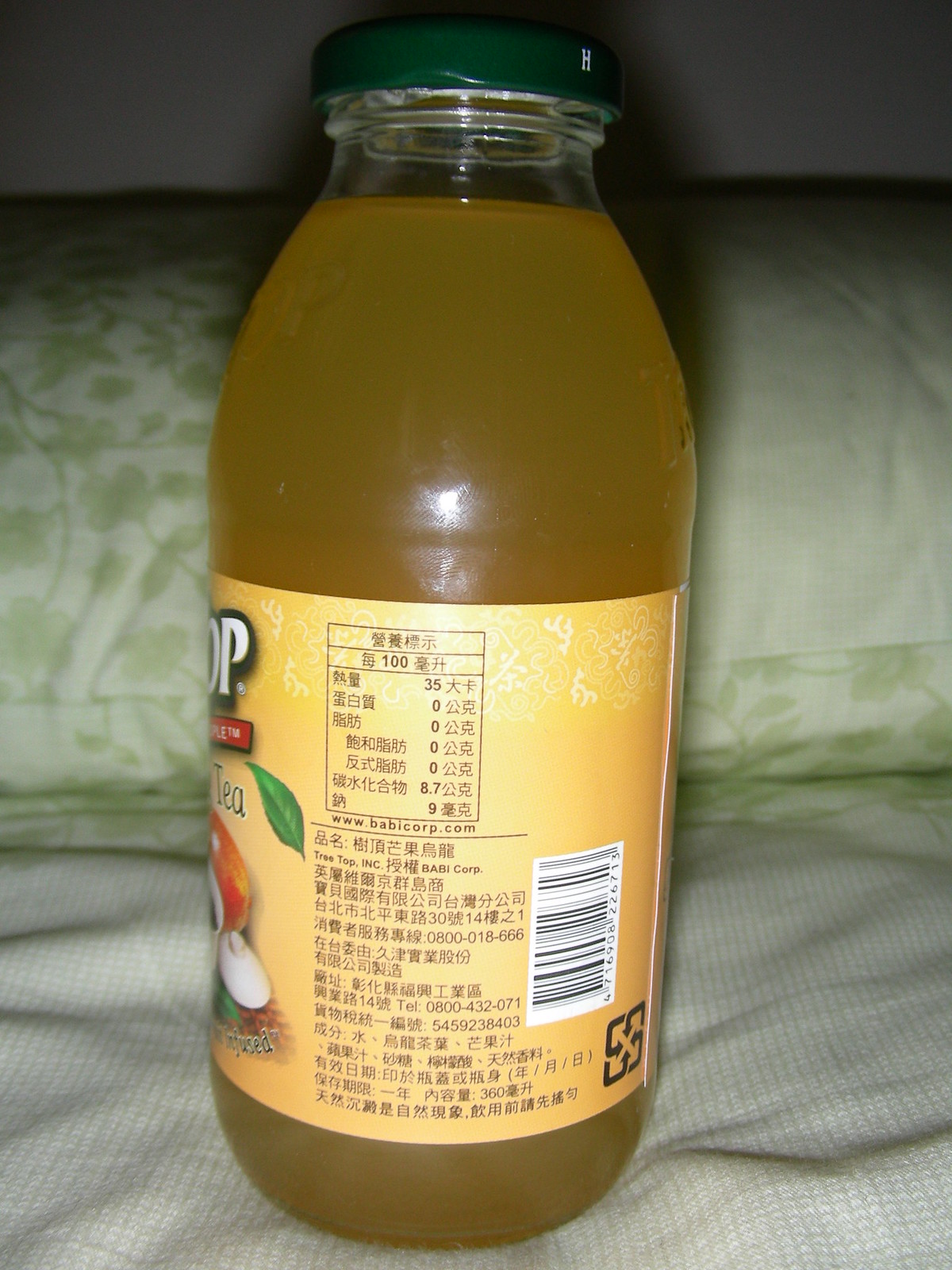This photograph features a neatly-arranged bed with a white fabric blanket and a green and white floral-patterned pillowcase. Dominating the foreground is a glass bottle of tea, distinguished by its dark yellow liquid and a green metal cap. The tea, identified as apple-infused, comes in a jar with a yellow label adorned with a well-known apple logo. The label has detailed nutrition information in an Asian language, most likely Chinese or Japanese, and prominently displays the text "tea" in English. Additional details on the label include a barcode, a recycling symbol, and the website "www.babbycorp.com." There are also numerical values like "100," "35," "8.7," and "9," which are part of the nutrition information, along with the word "infused." An image of peeled apple slices reinforces the apple theme of the tea. Overall, the scene captures the cozy setting of the bed juxtaposed with the inviting bottle of apple-infused tea.